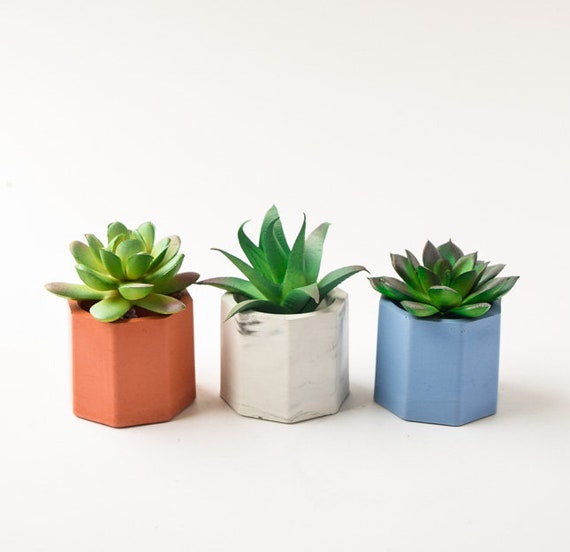The image features three octagonal-shaped planters, each containing a different succulent plant. The planters are displayed in a white environment, set on a white surface with a white background. The first planter on the left is an orange-colored pot housing a succulent with thick, oval-shaped leaves that fan out like a lotus, with some ends exhibiting a beige mauve hue. The middle planter is a white marbled pot that contains an aloe-like succulent, which is mostly green with some mauve-colored tips on its leaves. The planter on the right is baby blue, featuring a succulent with dark gray leaves that have green undersides. The light source is coming from the left, highlighting the textures and colors of the plants and planters, which appear to be crafted from either clay or plastic, with the middle one showing possible handmade characteristics.